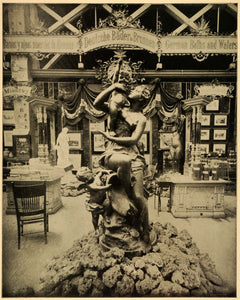The image is an old, black-and-white photograph, yellowed with age, capturing a detailed view of a statue in a seemingly historical or museum setting. The statue appears to depict a woman, possibly an allegorical figure, reminiscent of a mermaid or a maternal figure holding a child who reaches into the air. She wields a staff or blade in her arm, gazing upwards. The statue is elevated on a textured, non-symmetrical pedestal that resembles organic formations like large leaves or rocks. Surrounding this setup, there are various background elements including a balcony with unreadable banners, three distinctive X's against a dark backdrop, and a setting suggestive of a market, restaurant, or museum with tables, chairs, and numerous displays. The floor has a standard patterned design, though it is not clearly visible due to the photograph's faded condition.